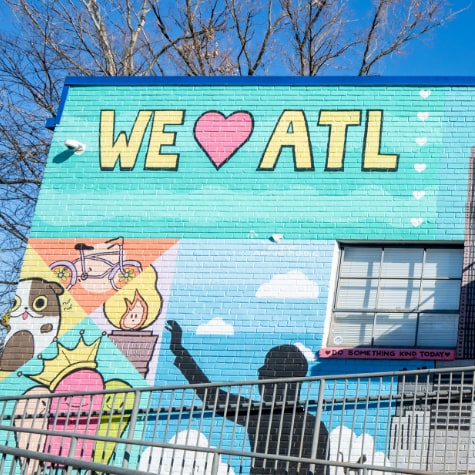The image depicts the side of a brick building adorned with detailed, colorful artwork. The upper section of the wall features a bold sign painted on a bluish-green background with the words "WE ❤️ ATL" in large yellow letters, where the heart symbol is pink with a black outline. Surrounding the text are six small white hearts and a dark blue border at the top. Below this, an artistic mural spreads across the facade.

In the center of the mural is a light blue sky with scattered white clouds, creating a serene backdrop. To the left of the main text, a security camera is visible, seemingly part of the building's infrastructure. Various illustrated sections populate the rest of the mural, divided into distinct quadrants.

One upper quadrant depicts a white bicycle against an orange background. Another quadrant shows a fire with a white core and a yellow outline against a purple background. Below these, the third quadrant displays three sausages, the middle one adorned with a crown and painted red. The last quadrant illustrates a fat, white dog with brown spots on a lighter tan background. Interspersed throughout this section are additional playful elements: a figure of a silhouette of a person reaching up and the suggestion of a fat dog character.

Adjacent to the building, a railing indicates a downward ramp, adding to the scene's depth. Behind the building, a bare tree stretches into a clear blue sky, grounding the vibrant urban artwork in its natural surroundings.